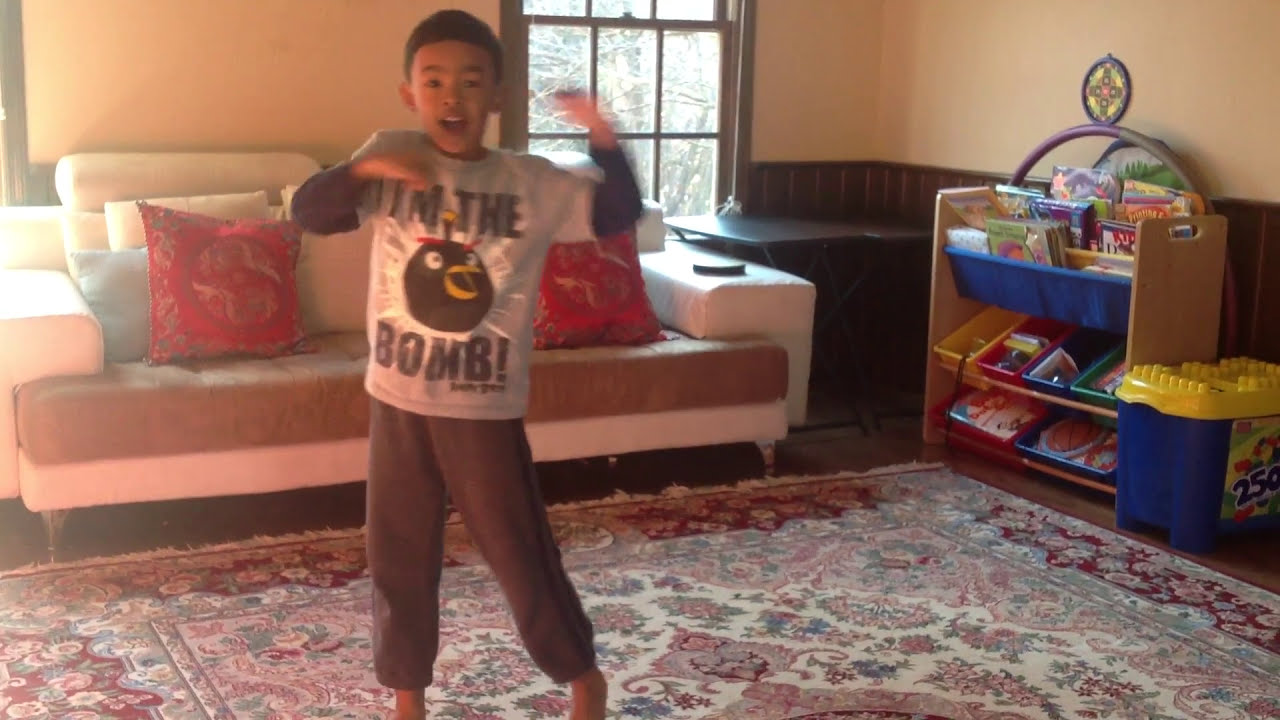In a brightly-lit living room, a young boy, around six or seven years old, joyfully stands at the center, seemingly caught mid-dance with his arms enthusiastically extended upward. He wears a light gray shirt adorned with a character from the Angry Birds video game and the text "I'm the bomb," and gray sweatpants, both complemented by a pair of darker colored long sleeves underneath the shirt. His thin, black hair frames his excited expression as he smiles directly at the camera.

The boy stands barefoot on a large Persian rug that combines burgundy, white, and other intricate patterns. Surrounding him, the room features a mix of brown wooden molding along the lower half of the cream-colored walls. To his right, there's a wooden shelf equipped with colorful buckets in blue, red, yellow, and green hues, filled with children's books and toys. Adjacent to this is a storage container labeled "250" containing blocks.

Behind the boy, a white leather couch peeks into the frame, adorned with an assortment of pillows. A window sits at the top center of the image, further illuminating the scene, and adding to the daytime ambiance of this cozy, playful space.